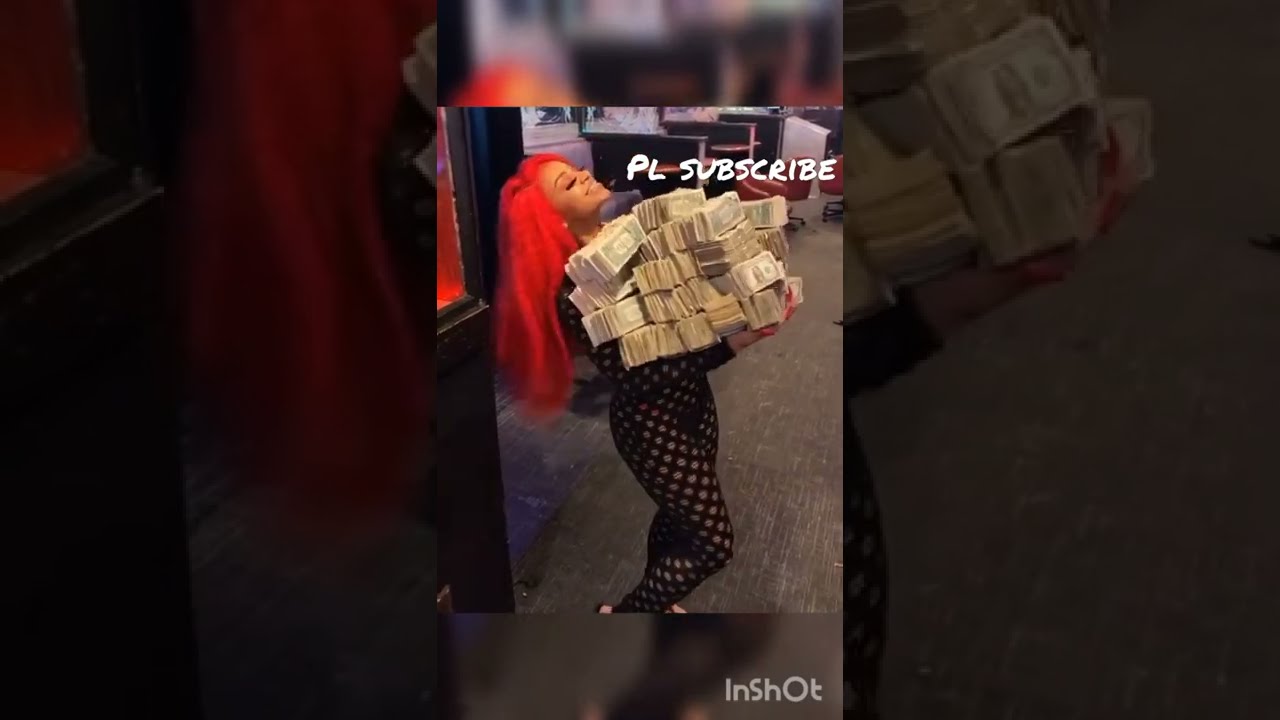The image is a highly detailed composite photograph with a central brightly-lit portrait flanked by two enlarged and darkened zoomed-in sections of the same image. At the heart of the composition is a young woman with vivid, long red hair cascading down her back, potentially hair extensions. She is clad in a striking black and white checked bodysuit that covers her from neck to feet. Her artificial long red nails are visible as she carries numerous bundles of $1, $10, and $100 bills, with at least 20 bundles stacked in her arms, which appear heavy. The woman tosses her head back, smiling with her eyes closed as she moves. Above her on the right side, the image features the text "PL subscribe, please subscribe" in white lettering, while the lower right corner displays the logo "INSHOT" also in white. The background hints at either an office space with chairs on wheels and booth-like structures or potentially a movie set, adding an intriguing spatial context to the overall image.